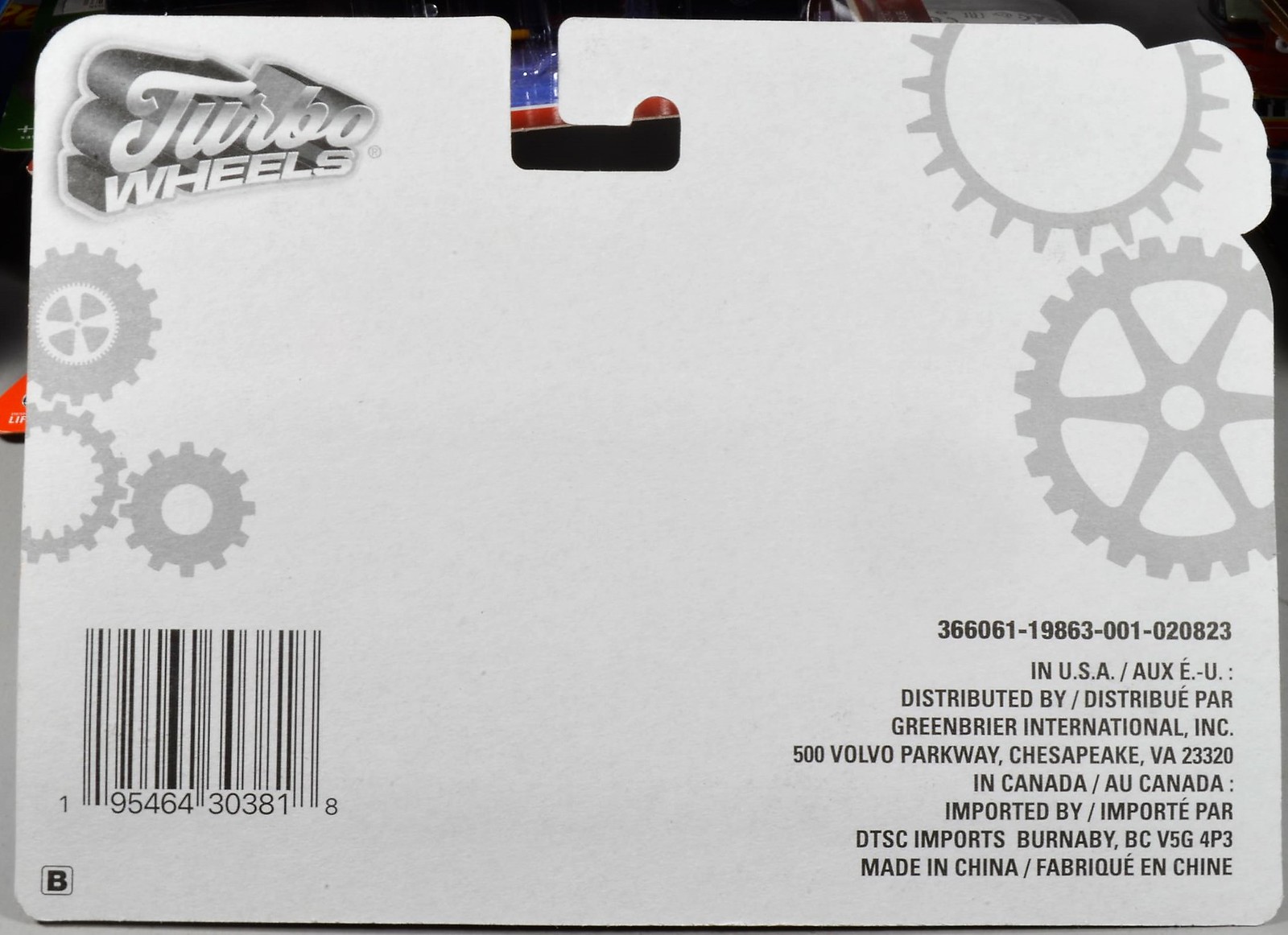This image features the back of a toy packaging, specifically for a product branded "Turbo Wheels." The cardboard backing displays a vibrant and eye-catching design. In the upper left-hand corner, the "Turbo Wheels" logo stands out with its 3D white and gray lettering. Surrounding the logo are several outlined gears: a cluster of three smaller gears directly beneath the logo on the left, and two larger gears positioned in the upper right section of the packaging. 

At the center top, there is an oval cutout designed for hanging the package on a retail hook. 

The bottom left-hand corner contains a barcode labeled with the numbers "9546430381" positioned in the center of it. To the left and right of the barcode, numbers "1" and "8" appear respectively. 

In the bottom right-hand corner, there is another series of numbers: "366061-19863-001-020" followed by "0823" in bold black letters.

Accompanying text provides manufacturing and distribution information. It reads: "Distributed by Greenbrier International, Inc., 500 Volvo Parkway, Chesapeake, Virginia, USA." Additional language indicates the product’s distribution in Canada and includes a French translation. The text also specifies that the item was "Made in China."